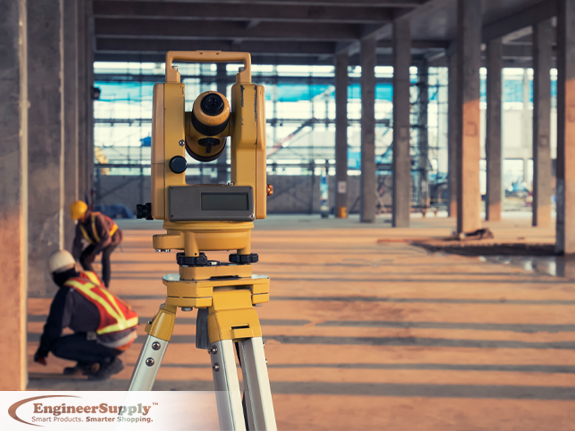This is a detailed photograph of a construction site dominated by surveying equipment, prominently positioned on a silver tripod with a yellow base. The equipment features a yellow rectangular frame with a cylindrical yellow tube and black stripes centered between two yellow handles, pointed towards the viewer. The scene is set against a blurred background illuminated by an orange hue, revealing a mix of pavement or dirt surfaces.

Tall gray concrete pillars cast their shadows across the construction site floor and stretch up towards a ceiling traversed by concrete beams. Dark scaffolding adorned with blue tarps is visible in the distance, hinting at ongoing construction activities. In the bottom left corner, two construction workers in high visibility vests—one in a white helmet and the other in a yellow helmet—are seen crouching, possibly engaged in measurement tasks.

Additionally, the bottom left features a white gradient triangle emblazoned with a brown ARC logo and the text "Engineer Supply Smart Products Smarter Shipping." The overall image composition is rectangular, wider than it is tall, providing a comprehensive glimpse into the structured, industrious environment of the construction site.